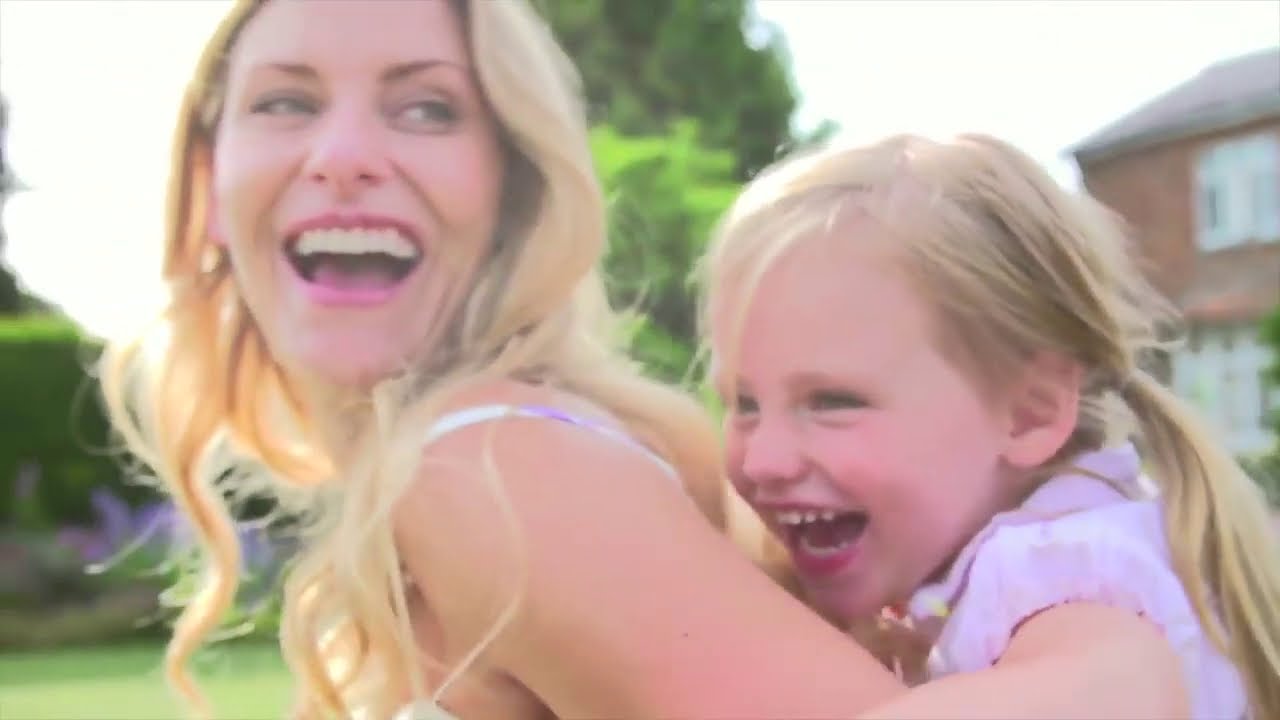The image is a close-up, shoulder-up photograph of a smiling mother and her young daughter, set outdoors in what appears to be their suburban front or backyard. The mother, who looks to be in her thirties, has long, wavy blonde hair and is wearing a light purple spaghetti strap tank top that tapers into a white color at the front. She is looking over her left shoulder at her daughter with a joyful expression, her mouth open in laughter. The daughter, perched on her mother's back, appears to be around three years old and has blonde hair tied in pigtails. She's wearing a light pink shirt and also has her mouth wide open in a happy smile, looking straight ahead. Surrounding them are green lawns and large trees, with a glimpse of a red brick house with a gray roof and white-trimmed windows in the background. The bright, sunny day enhances the vibrant colors of the scene, including touches of gold in their hair and shades of green and brown from the foliage and house, respectively.